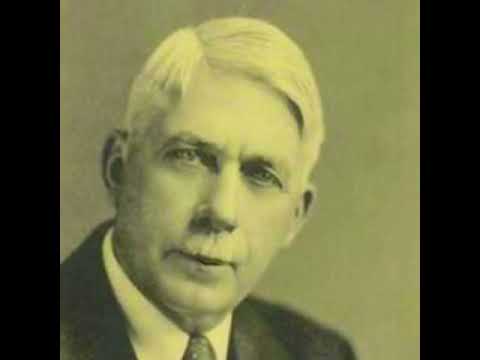The image depicts an antique black-and-white portrait of an older man, likely from the 1910s to 1920s. The photograph exhibits a unique greenish-yellow hue, enhancing its vintage appearance. The man has white hair neatly combed to the side and a narrow, white or gray mustache, giving his fair-skinned features a distinguished look. He is dressed in a dark suit jacket, a white button-up shirt, and a necktie, possibly black though the color is unclear due to the photo's tint. His head is tilted slightly, with a quizzical, neutral expression, and his face is centered while his body is cut off at the shoulders. The plain background, likely part of a photographic studio setup, has a beige tone bordered by two black bands on the sides, lending the scene a formal air reminiscent of corporate or family portraits intended for display.